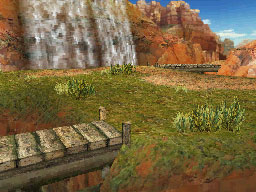This vibrant color image appears to depict a scene from a computer game. In the foreground, situated in the bottom left-hand corner, there is a structure that resembles a wooden or stone plank pathway. The pathway consists of rectangular slabs interspersed with patches of green grass or weeds.

Adjacent to this pathway are areas of orange ground and more green grass, dotted with small shrubs. Moving towards the background, the orange terrain extends further back. 

On the left side of the image, a towering mountain or cliff face made of grey rock looms prominently. A section of reddish rock is visible in both the left-hand corner and the center-right, adding a unique contrast to the scene. 

The cliff edge appears to drop off towards the right corner of the image. The sky in the background is a clear blue, adorned with scattered clouds, enhancing the picturesque quality of the landscape.